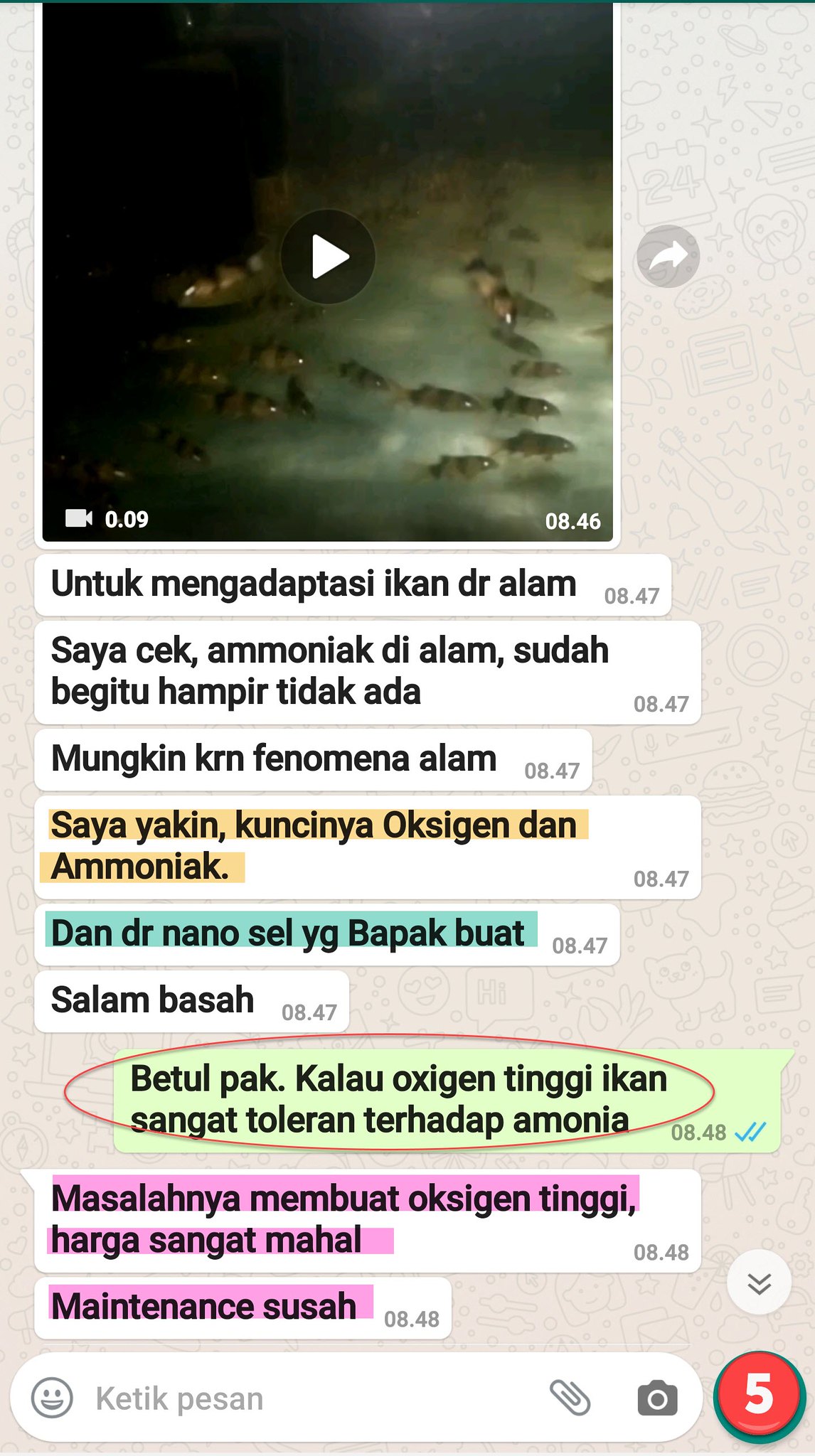The image appears to be a screenshot from a smartphone application, likely a messaging app, and features a video thumbnail at the top depicting an aquarium or murky water with a school of brown and black striped fish. The thumbnail includes a white play triangle, indicating it is a video, along with a video icon at the lower left corner showing '9 seconds' and a timestamp of '8:46' at the lower right corner. Below the video, numerous white text bubbles, highlighted with various colors such as green and purple, are present. The text within these bubbles is written in a foreign language and includes phrases like "Antuk Mengadaptasi Ikan Daktar Alarm Alam" and "Betul Pakalu Oxygen." There are various timestamps like '8:47' and '8:48' associated with these comments, suggesting a sequence of messages or annotations. At the bottom of the screenshot, there's a chat input bar with an attachment icon and a red circle indicating '5' unread messages, hinting at active conversation within a group chat context.